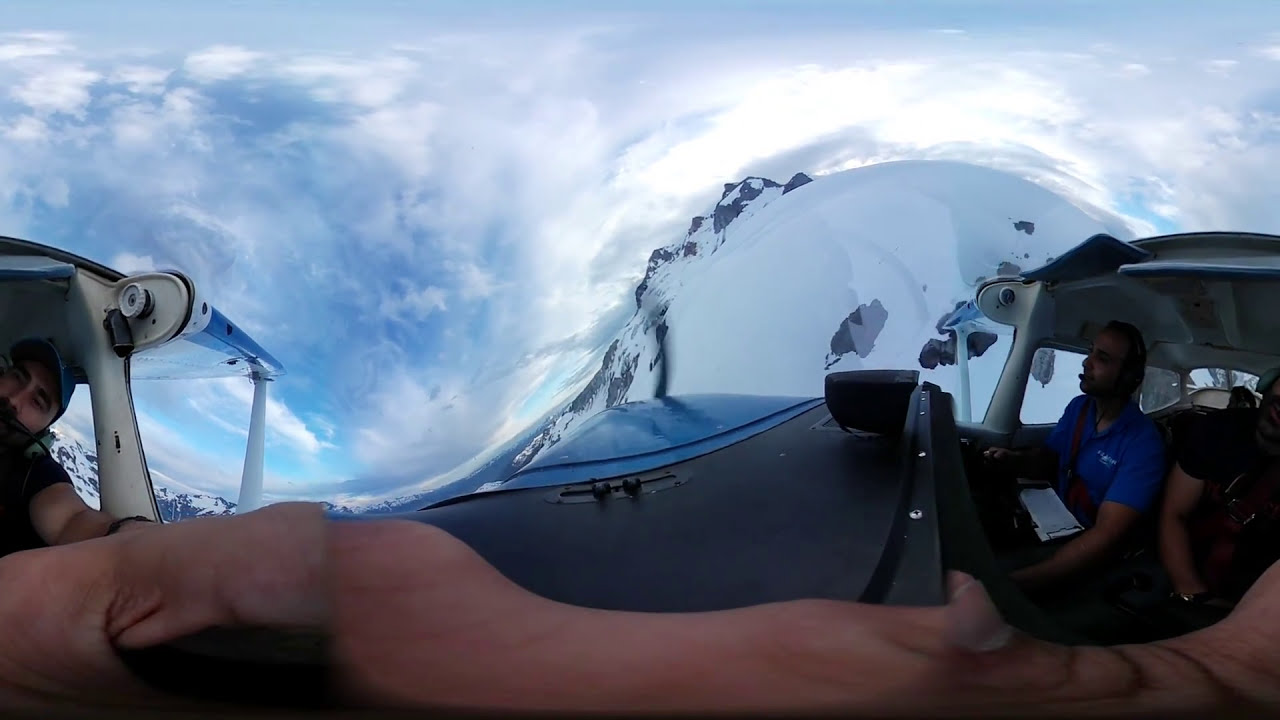The image, a highly distorted and surrealistic photograph, captures the interior of a plane or some sort of vehicle in flight. The scene, presumably taken with a wide-angle lens, features both the passenger and cockpit views, showing a Caucasian man in a blue ball cap and green over-the-ear headphones on the left. His hand extends unnaturally across the entire width of the photo, morphing into a fleshy mass that merges with another person's hand on the far right, who is a brown-skinned man in a blue short-sleeved polo shirt, possibly the pilot.

Above this bizarre merging of limbs, the sky is a mishmash of stitched images, with the blue sky and white clouds forming a concave dip on the left, rising up into a mountain-like shape in the center, and flowing out again on the right. The landscape below is a snowy mountain range, adding to the overall oddity of the captured scene. The background reveals a twisted and contorted blue sky, blending with the tops of mountains, which juts out in unusual circular shapes, creating an eerie backdrop to the interior chaos of the vehicle. The amalgamation of these strange elements results in an image where reality mingles with the bizarre.